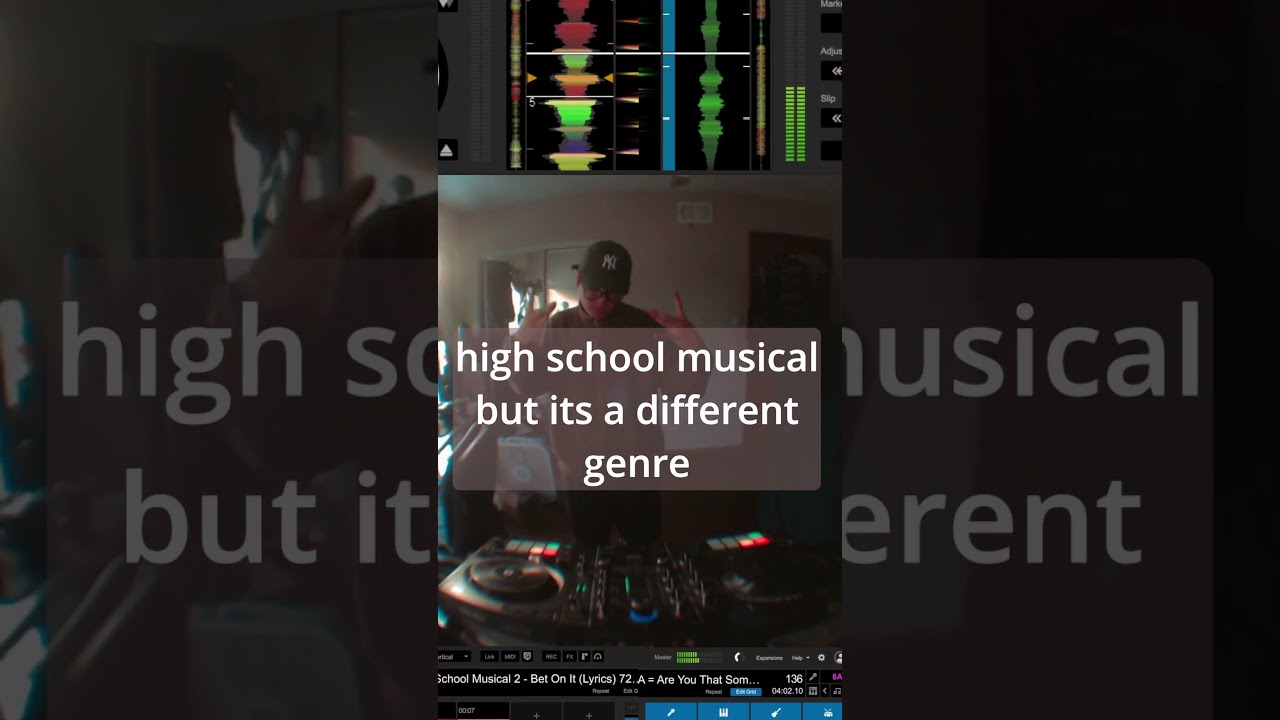The vertical cell phone-style photograph features a young Asian disc jockey standing in a room with a light-colored wall, flanked by a window on the left and a doorway on the right. The main image, which is centrally positioned and bordered above and below by various scenes of digital audio equipment, shows him wearing a dark gray New York Yankees cap and glasses, and dressed in a black jacket. He stands before a black turntable adorned with numerous knobs and red, green, and orange lights, with his hands raised and fingers splayed out as he looks down at his equipment. Superimposed on the bottom half of the image is semi-transparent white text divided into three lines, reading, "high school musical but it's a different genre". The image itself is framed on both the left and right sides by zoomed-in, faded versions of the same picture, creating a grayed-out border effect.